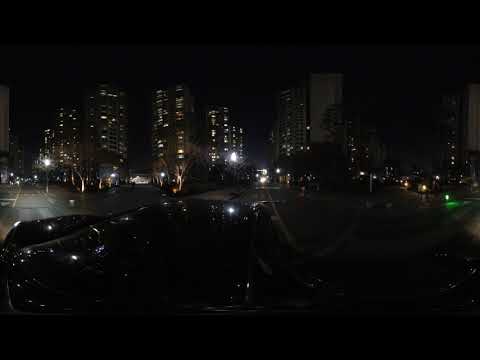In this nighttime photograph, the scene presents a striking view from inside a sleek, black, Batmobile-like car driving through what appears to be the bustling streets of New York City or another major city. The dominant color is black, emphasizing the nighttime setting, with the sky clear but devoid of any visible stars or the moon. The reflection of city lights glistens on the shiny surfaces of cars, hinting at their sleek, dark exteriors.

The foreground is dominated by a roadway lined with parked vehicles, their outlines softened by shadows. The midground features crosswalks, numerous streetlights, and an array of city elements such as traffic lights and stop lights that cast their own hues of green and yellow, adding dynamic splashes of color to the scene. Tall buildings, likely residential towers standing roughly 20 stories high, form the backdrop, their windows sporadically lit by the warm glow of interior lights, indicating inhabited apartments or condos.

To the left, a dimly lit avenue and a bright street lamp highlight an intersection, while on the right, a faint green traffic light marks another unseen crossing. The image exudes a sense of motion and possibility, as if one could venture down multiple routes branching off this main road, exploring the unique blend of urban and potentially countryside elements suggested by the surroundings. This detailed composition effectively captures the vibrant and multifaceted essence of night in a grand cityscape.